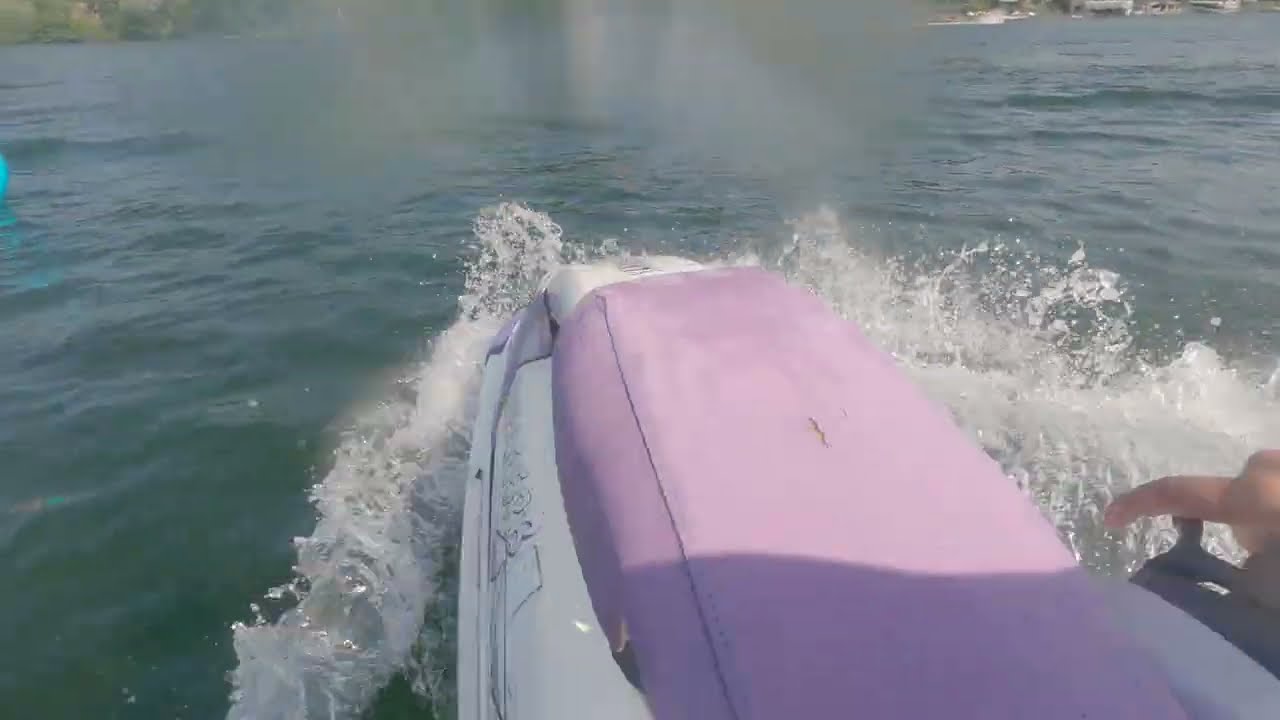The photograph captures a close-up, rear-view scene of an individual jet skiing on a lake. The image prominently features the jet ski's handlebars, which have light purple foam grips and black hand gears. The rider's hands grip the handlebars, with a blue curly cord, resembling a telephone cord, possibly attached to the key or the driver for safety. The white frame of the jet ski, adorned with instructional and warning stickers in orange and black text, is visible at the bottom center of the photograph. The body of water reveals ripple patterns and waves, with the shoreline visible in the distance, bordered by trees and some distant structures. The sky appears partly cloudy, providing a natural, outdoor daytime setting. The overall color palette includes shades of lavender, blue, green, white, black, red, tan, and gray. There are no other people, boats, or evident fish in the water, emphasizing the solitary nature of the jet skiing experience.